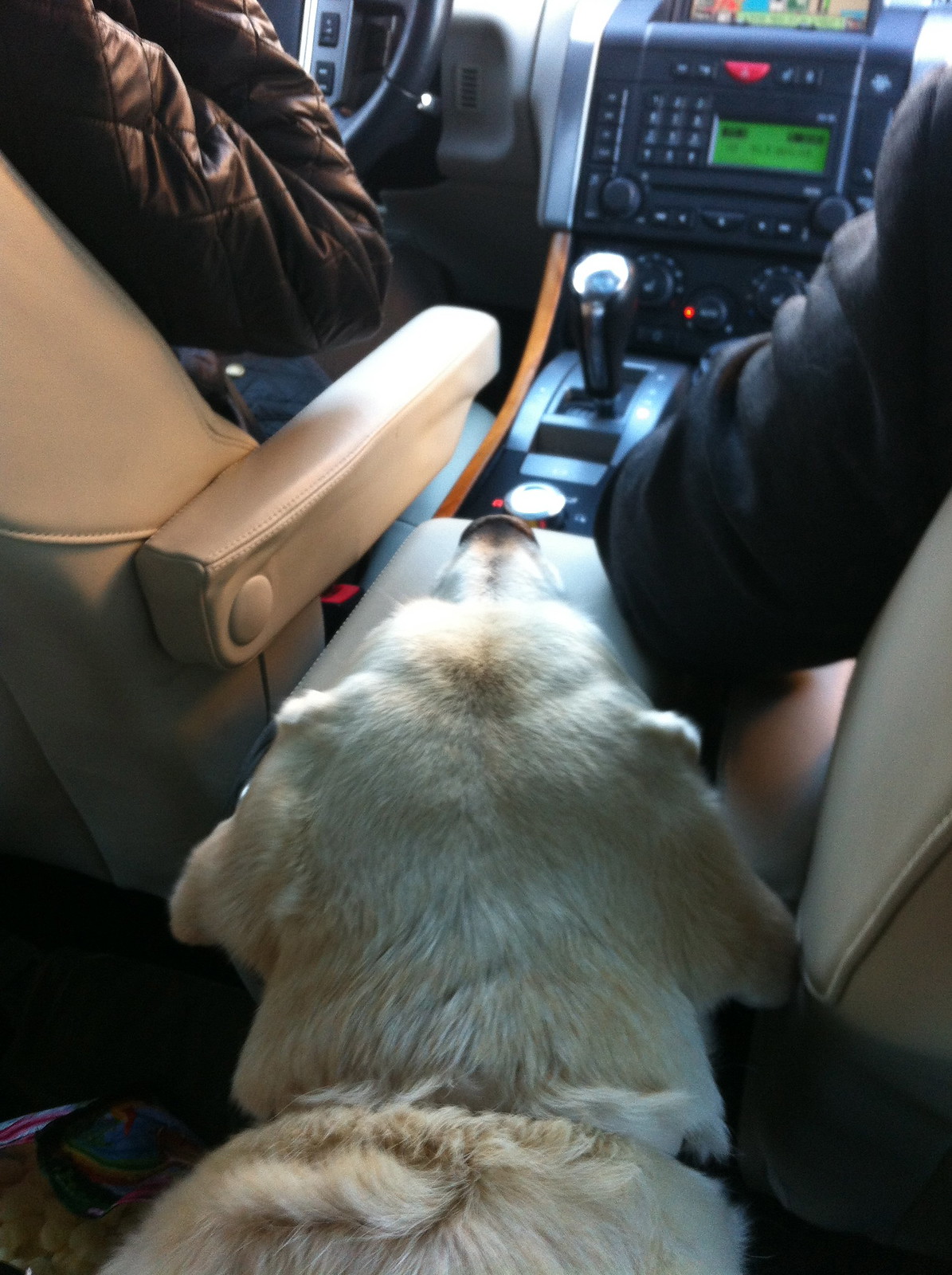The photograph captures a cozy scene from the vantage point of someone sitting in the back seat of a car. In the foreground, a blonde-colored dog, likely a golden retriever or labrador mix, with drooping ears and a small, visible part of its collar, rests its head endearingly on the center console. This console, matching the tan leather or faux leather upholstery of the front seats, is nestled between two foldable armrests that are down. The driver's brown padded jacket and the front passenger's black jacket are clearly visible. The driver's right arm is bent upward at the elbow, while the passenger's arm rests on the console. Detailed elements of the car's interior, like the gear shift, various buttons, black knobs, steering wheel, and two screens on the dashboard, add to the depth of the scene. The shared tan upholstery, subtle reflections on the leather surface, and the dog's relaxed posture contribute to a warmth and intimacy in the image, illustrating the silent bond between the passengers and their faithful canine companion.